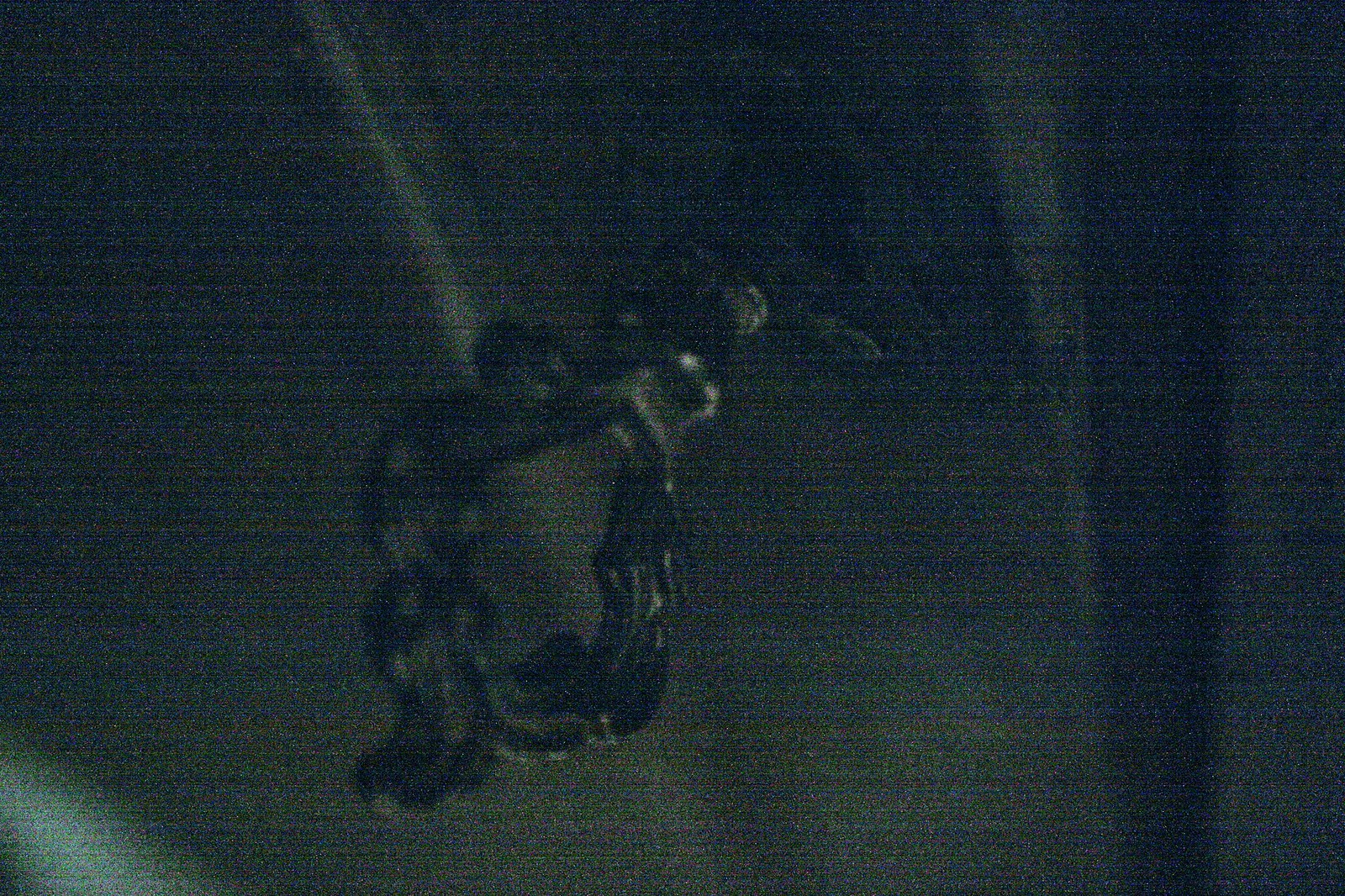This very close-up and slightly blurry photograph centers on a drawer pull attached to the front of a drawer. The drawer pull features a distinct design. At the attachment point, there's a light-colored metal circle. Extending from this circle is a black metal piece that forms the main handle. The handle itself is oval-shaped with indented edges, breaking away from straight lines to create a more intricate pattern. The middle of the handle is completely open, forming an empty space, and at the bottom, there is a small tail-like extension curving to the left. The drawer pull is made of thick black metal. The drawer to which it is attached can be seen in the background, but it is significantly faded and out of focus, making the drawer pull the prominent element in the image.